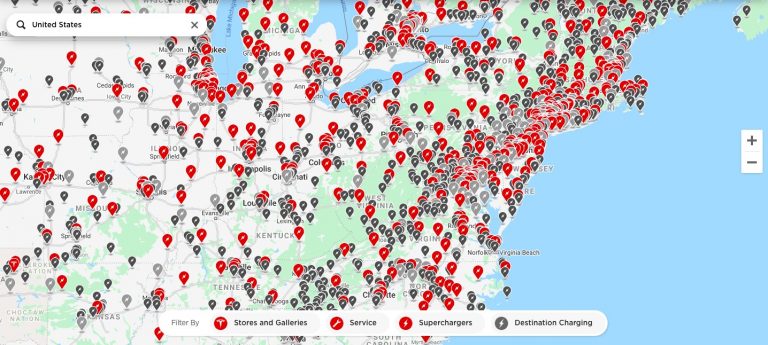This image depicts a detailed section of a map of the United States. The map is displayed within a long rectangle stretching from left to right. In the top left corner, "United States" is written in blackish-gray text inside a search bar. The map is peppered with numerous red and gray balloon markers, too many to count, representing various points of interest across the country. 

On the right side of the map, a blue area signifies the ocean. Below the map, at the bottom center, there's a "Filter by" label followed by multiple icons. The first red circle represents "Stores and Galleries," followed by another red circle indicating "Service." Next is another red circle with an image, labeled "Superchargers," and lastly, a gray circle featuring a lightning bolt, marked as "Destination Charging."

The map also highlights specific states, with labels for West Virginia and New York being visible.